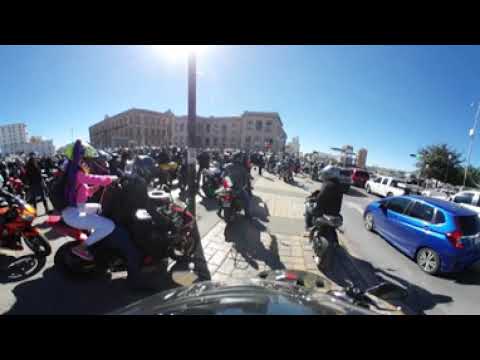The rectangular photograph, framed with solid black bars across the top and bottom, depicts a lively street scene bathed in clear, sunny sky without a cloud in sight. Dominating the image, numerous people are gathered around and on motorized scooters, suggesting a possible group ride or event. Prominently on the left, a woman wearing white pants, a pink shirt, and a neon green helmet is seen holding onto a man on a motorcycle. In the center, a dense collection of scooters showcases riders all wearing helmets. To the right, a variety of vehicles, including a bright blue compact car, a red van, and a line of trucks, are visible. The road beneath them is a mix of asphalt, pavers, and concrete. The background is adorned with large, multi-story buildings in off-white hues, punctuated by numerous windows and openings, adding an urban context to the scene.